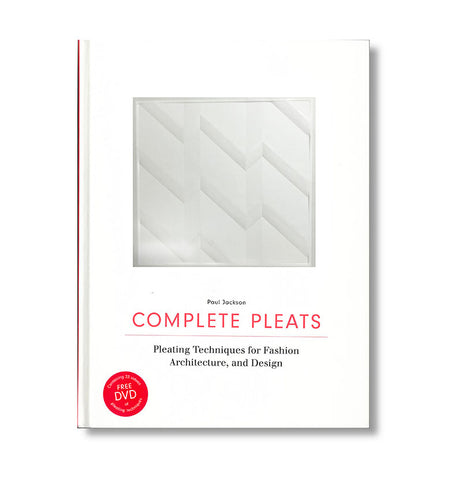The image depicts the cover of a hardcover booklet titled "Complete Pleats" by Paul Jackson. The cover is predominantly white, featuring an intricate pleated design that resembles folds of cloth or architectural pleats. The title "Complete Pleats" stands out in large, bold red capital letters, while the subtitle "Pleating Techniques for Fashion, Architecture, and Design" is written in black beneath it. Above the title, the author's name, Paul Jackson, also appears in smaller black text. In the bottom left corner, there is a prominent red circle with the words "Free DVD" in white text inside it, although the smaller text around the edge of the circle is too blurry to read. The cover's clean design and clear text suggest it's a comprehensive guide on pleating techniques across various disciplines.